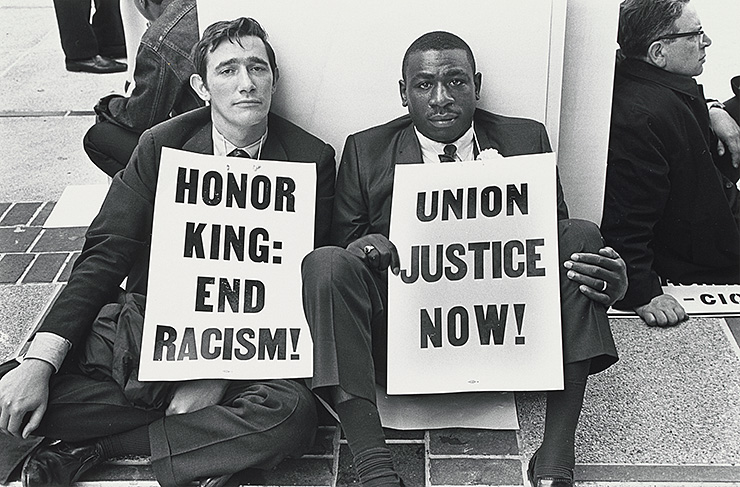In this evocative black-and-white photograph, likely captured during the Civil Rights era, a powerful scene unfolds around a central white pillar. The floor is lined with red tiles, possibly granite cement, and the setting appears to be a public space such as a street or subway station. At the heart of the image, two men—a black man and a white man—sit side by side on the ground, leaning against the pillar. Both are dressed in black suits, white shirts, and black ties, and each wears a wedding ring. They hold signs around their necks, broadcasting poignant messages: the black man's sign reads "Union Justice Now!" while the white man's sign advocates "Honor Dr. King! End Racism!" Flanking them, other individuals also lean against the pillar, suggesting a sit-in protest. In the background, additional protesters are visible, including a person standing in the top left corner, heightening the sense of collective solidarity and action.